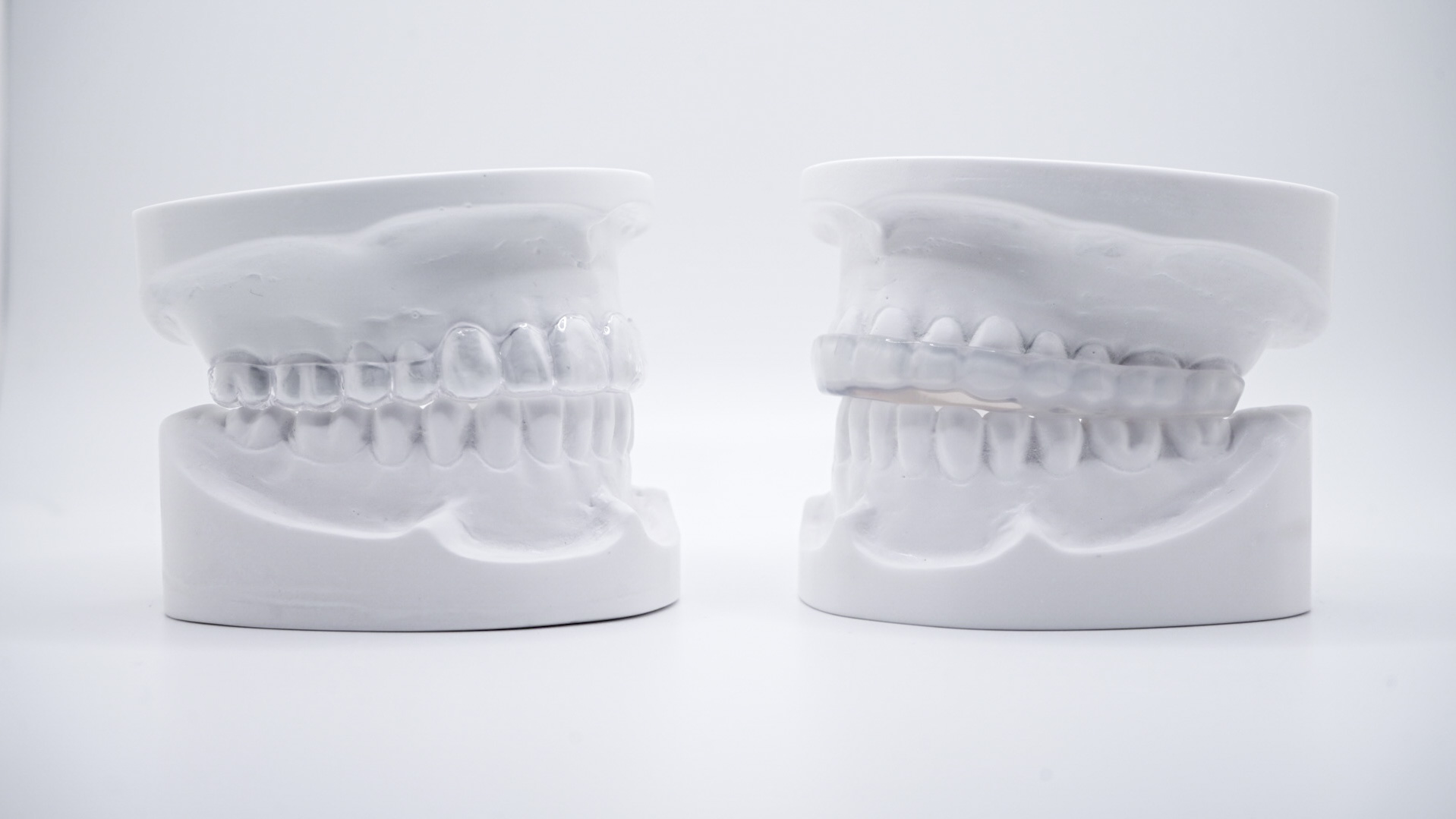The image showcases two detailed dental models placed on a white surface with a plain white background, presenting a clinical and clean aesthetic. Both models feature upper and lower jaws with realistic sculpted teeth and gums. The model on the left is equipped with a contoured, nearly invisible dental brace reminiscent of Invisalign, designed to fit over each tooth seamlessly. In contrast, the model on the right displays a bulkier, see-through plastic mouth guard that envelops the upper teeth, possibly serving as a retainer or protective cover against overbites. The dental appliances highlight different orthodontic treatments, and the models are positioned to face each other, providing a clear view of each type of dental aid.